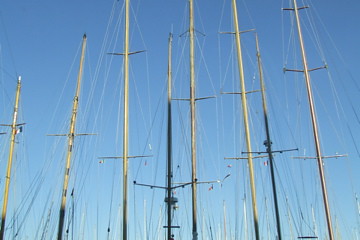This color photograph captures a beautiful, clear, and cloudless blue sky as the backdrop. Dominating the foreground are the masts of multiple ships, with each mast resembling long, slender poles extending vertically into the sky. There are eight such masts in the image, and they appear light in color, potentially wood, with darker hues towards the base. A notable detail is that one mast in the center seems to have some sort of electronic device or camera mounted on it. Suspended from the tops of these masts are numerous light-colored wires or cables, which extend downwards and seem to crisscross and intertwine, making it difficult to trace a single wire from beginning to end. The masts are aligned in a way that suggests the cables may link between adjacent masts. There are no additional elements in the photograph such as people, animals, plants, or vehicles, allowing the viewer to focus entirely on the intricate network of masts and wires against the expansive blue sky.